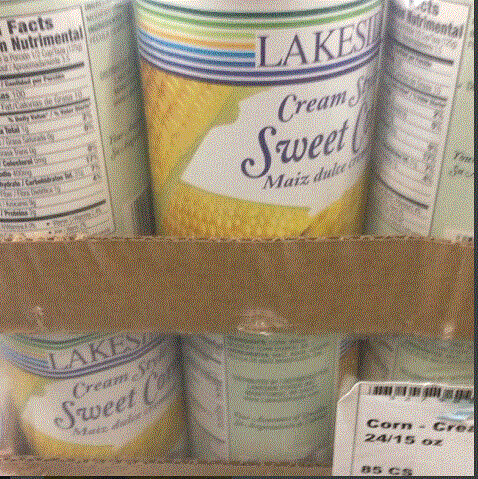The image captures two cases of Lakeside brand cream-style sweet corn, stacked in low-sided cardboard boxes wrapped in plastic, typically seen in grocery stores or wholesale locations like Costco. Each can features a white background label adorned with horizontal stripes in dark green, green, light green, orange, blue, darker blue, and purple, with the words "ocean sweet corn maize" in blue lettering. Prominent images of yellow corn dominate the label, with some cans turned forward and others sideways, exposing parts of the nutrition facts sticker and the product's branding. The lower right corner of the box displays a white and black sticker indicating "corn cream" and "24/15 ounces," indicating the case contains twenty-four, 15-ounce cans. The overall setting suggests a neatly organized product display in a retail environment, offering clear visibility of the corn products.